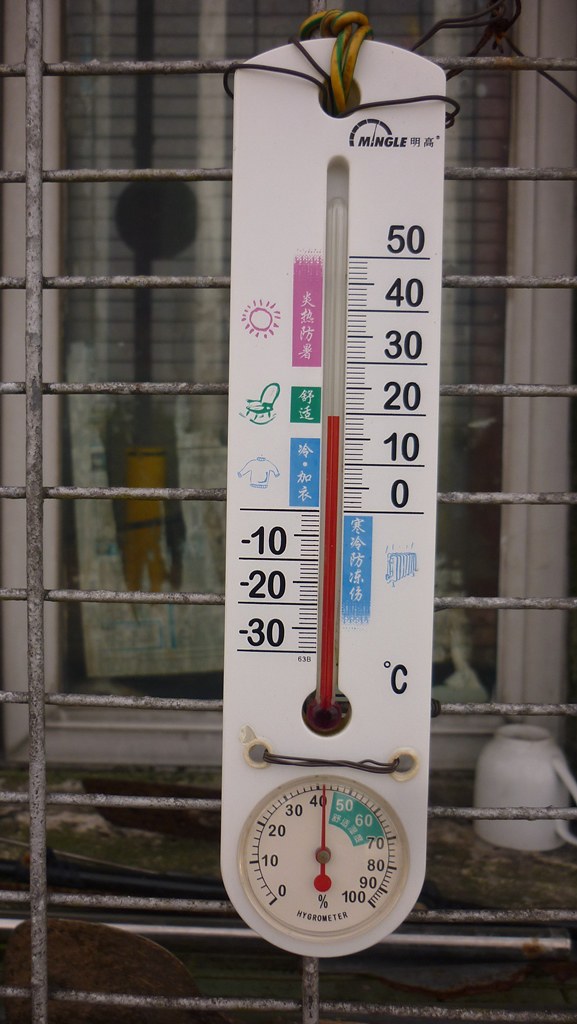This photograph captures a detailed scene involving a temperature thermometer firmly secured to a metal grill or lattice using black wire and a yellow cable. The metal grill is positioned against a window with a glass pane enclosed in a white frame. Resting on the window ledge is a white porcelain mug or teacup, adding a touch of homeliness to the image.

The thermometer itself is crafted from white plastic and features color printing, including an icon of a sun, a rocking chair, and a jumper. These icons provide visual cues for interpreting the temperature reading and suggest appropriate attire based on the weather conditions. The thermometer measures temperature in degrees Celsius, with a bright red liquid inside a glass tube currently indicating a temperature of 19 degrees Celsius.

Beneath the thermometer is a hygrometer, which displays the humidity level. The hygrometer, with its black-numbered dial, reads around 40-42% humidity. This reading is below the optimal humidity range indicated on the device, which is highlighted in a green pie-shaped segment between 45 and 68%. The optimal range generally falls between 50 and 60%, as suggested by the device.

This meticulously arranged photograph not only provides temperature and humidity readings but also subtly conveys the comfort and atmosphere of the setting with its thoughtful details.